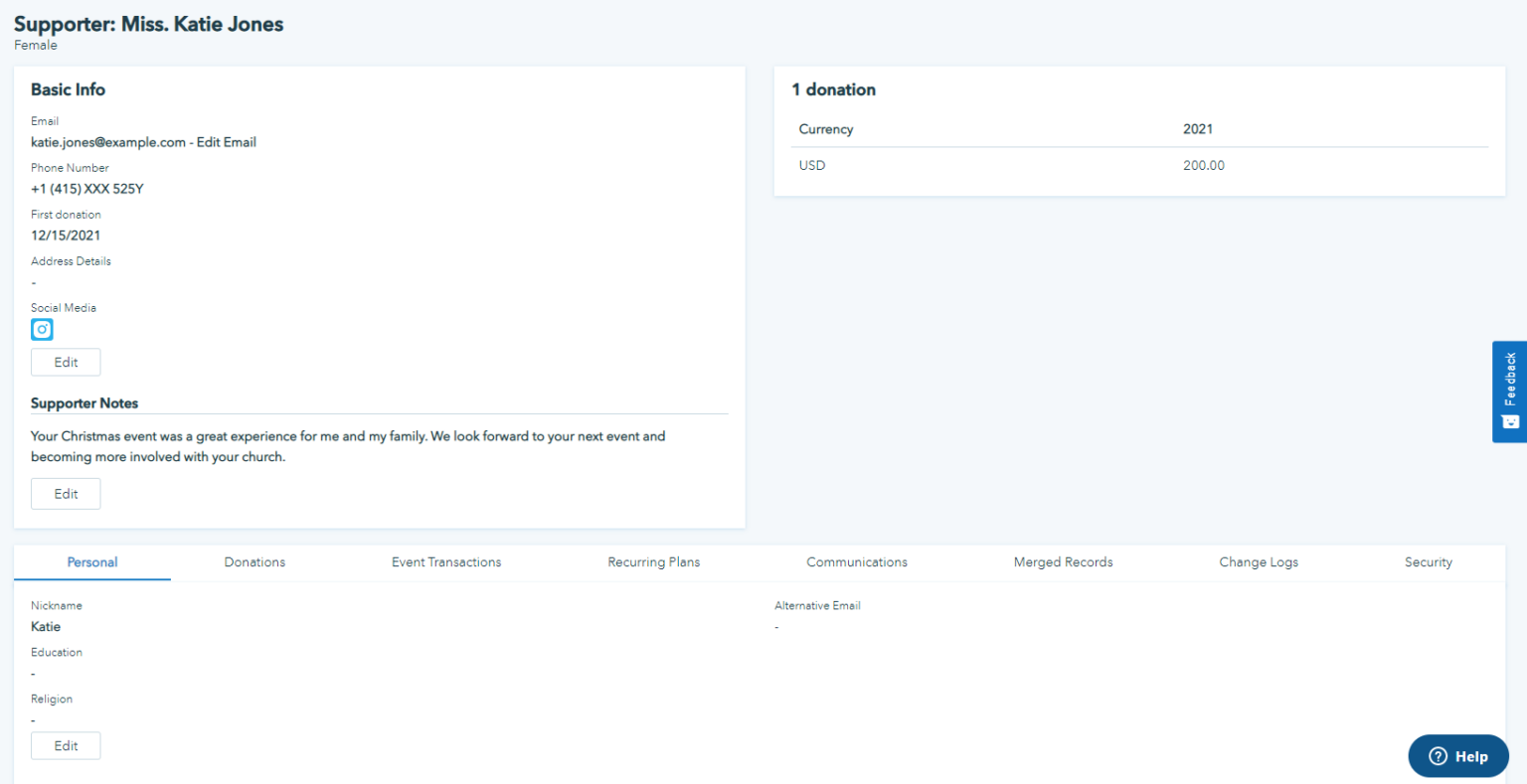The image is a horizontal screenshot featuring a detailed user interface with distinct sections and backgrounds. Dominating the design, a light gray background frames several white pop-up boxes. At the top left, a profile heading reads "Supporter: Miss Katie Jones, Female," immediately followed by a "Basic Info" box detailing Katie's email, phone number, first donation date, and address. An icon adjacent to this section provides a link to her social media page alongside an edit button for modifications.

Beneath the basic info, there's a "Supporter Notes" box filled with Katie's positive feedback: "Your Christmas event was a great experience for me and my family. We look forward to your next event and becoming more involved with your church," accompanied by another edit button for edits. To the immediate right, a compact horizontal box mentions "One Donation" in US dollars, specifying a $200 contribution made in 2021.

The lower portion of the screenshot features an organized header bar, with "Personal" highlighted in blue. Other clickable categories include "Donations," "Event Transactions," "Recurring Plans," "Communications," "Merged Records," "Change Logs," and "Security." The "Communications" tab reveals a note in small text stating "alternative email." Under the "Personal" section, selected on the left, it shows Katie's nickname, "Katie." The sections labeled “Education” and "Religion" are currently blank, with another edit button available for input.

In the lower right-hand corner, there is a prominent dark blue oval help button marked with a question mark and a circle icon, signifying user assistance functionality.